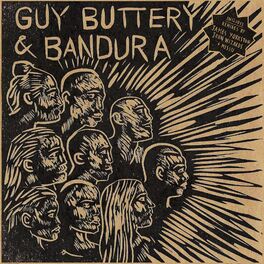The image appears to be an album cover featuring an artwork with a distinct, rustic aesthetic. The background is primarily black, providing stark contrast to the primary elements which are drawn in a combination of tan, brown, and gold hues. Central to the artwork is a group of seven or eight people, drawn sketch-style, whose heads and profiles face towards the right. These heads are arranged in the bottom left corner, and streaks emanate from them in a half sunburst pattern, giving an impression of radiating sound or energy, despite their mouths being closed.

At the very top of the image, the title "Guy Buttery and Bandura" is written in a handmade, rustic font. Additionally, in the upper right corner, there's a small star-shaped logo with some text inside that mentions "James York." The overall color scheme of the artwork is subdued yet striking, dominated by the interplay of tan and black tones.